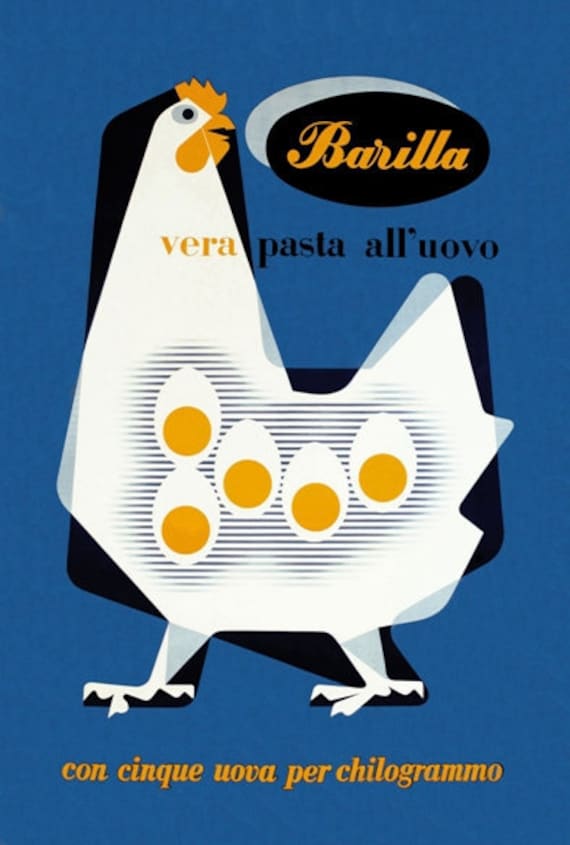This full-page, colored advertisement prominently features a cartoonish, white chicken set against a blue background with a subtle abstract shadow behind it. The chicken's head is tilted, and it looks to the right. Positioned within the chicken's belly are six boiled eggs, their white and yellow yolks clearly visible. The top of the poster displays a black circle with the word "Barilla" written in cursive, offset by a white ring behind it. Just below, the text reads "Vera Pasta al Uovo con Cinque Uovo per Kilogramo." Along the bottom of the poster, additional text in Spanish stretches across the length of the chicken.